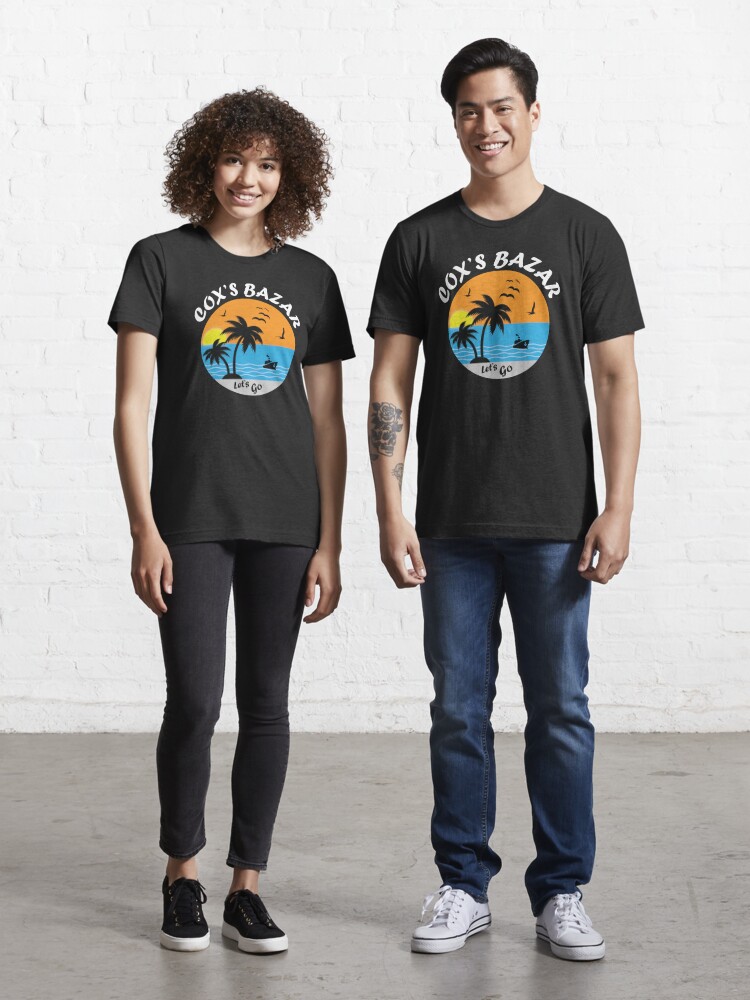In this image, a man and a woman are standing side-by-side against a white brick backdrop on a cement floor, both wearing identical black t-shirts with a colorful circular emblem featuring an orange sky, blue water, palm trees, and the words “Cox's Bazaar” above with "Let's Go" at the bottom. The woman, positioned on the left, has light skin, curly brown hair, and is smiling. She is dressed in black yoga pants and black sneakers with thick white rubber soles. The man to the right has short black hair, likely of East Asian descent, and a tattoo on his right arm. He is also smiling and wearing blue jeans and white sneakers with a blue striped bow on the sole. Together, they appear to be advertising their matching printed t-shirts.